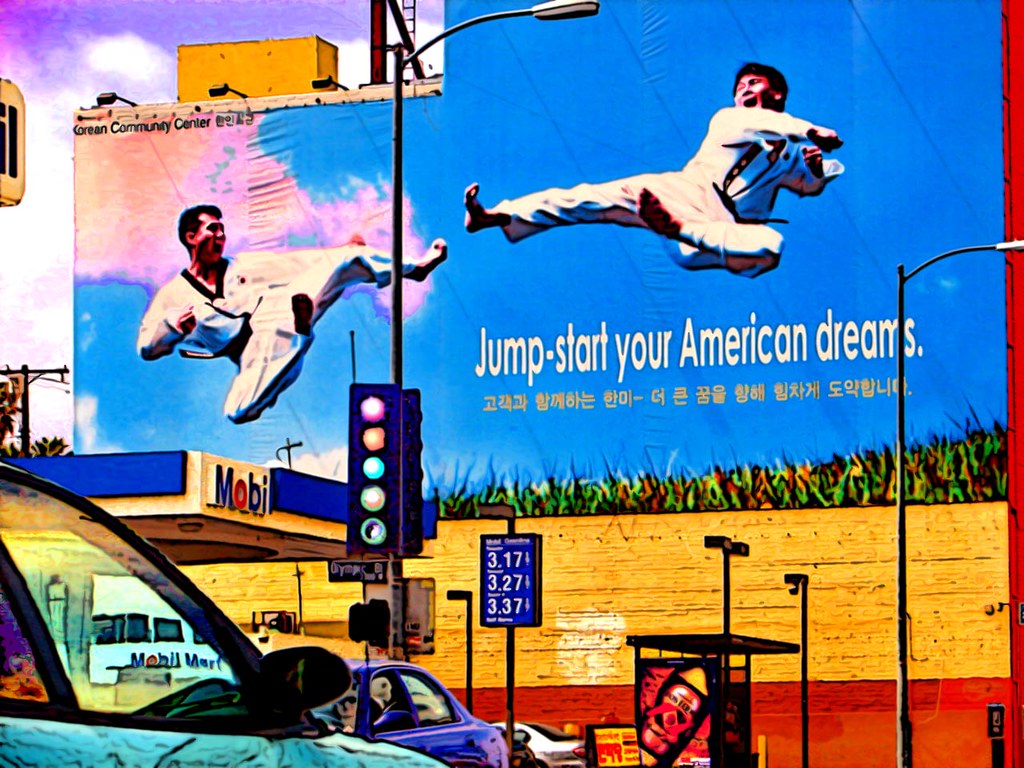The image depicts a digitally enhanced, colorful mural on the side of the Korean Community Center building. The mural features two Asian men in karate gear, frozen mid-air as they unleash dynamic kicks towards each other, their mouths open as if shouting. The background of the mural transitions from a cloudy blue sky at the top to green corn stalks at the bottom. Above the men, in the upper left corner, "Korean Community Center" is printed in black font alongside Korean text. Below the men, in bold white letters, it states, "Jumpstart your American Dreams," accompanied by Korean translation in gold lettering.

In the foreground, there is a busy street scene. On the left, a shiny blue car is stopped at a traffic light, with another dark blue car slightly behind it. The traffic light features a unique configuration with five colored circles: red, orange, green, yellow, and a green ring. Nearby, there's a blue and white Mobile Gas Station, with the sign reading "Mobi," with the 'O' in red. A mobile mart is visible within the gas station premises, displaying gas prices as $3.17, $3.27, and $3.37. Additionally, a black bus stop is positioned towards the right of the bottom center, and an old payphone, which appears to be painted onto the background, is in the right-hand corner. Overall, the image mixes both realistic and painted elements, creating a vibrant and surreal scene.